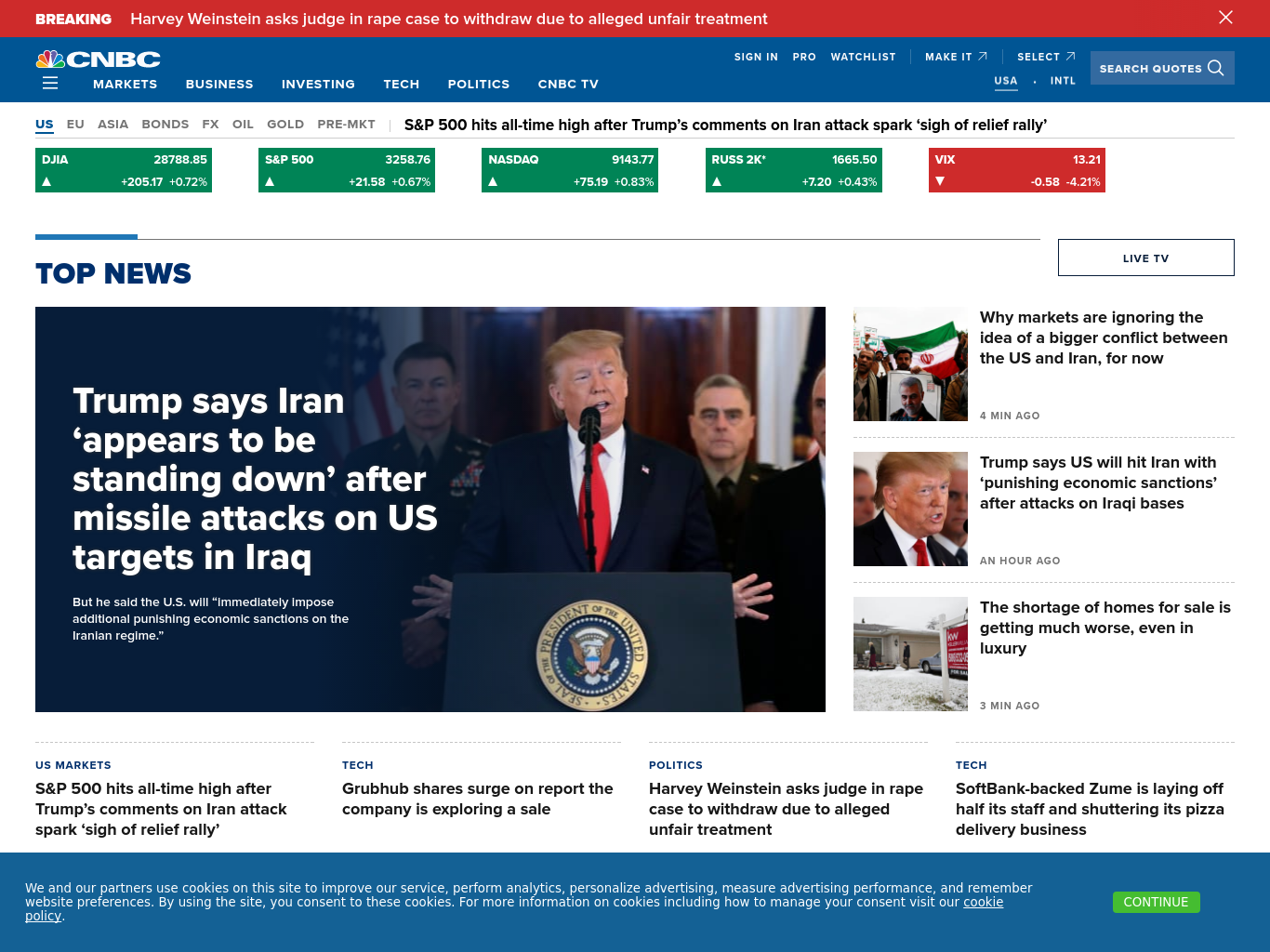This image is a detailed screenshot from the homepage of the CNBC website. The header is prominently blue, featuring the familiar NBC peacock logo on the left, followed by the white text "CNBC." Above the header, a red banner with bold, capitalized white text announces breaking news: "HARVEY WEINSTEIN ASKS JUDGE IN RAPE CASE TO WITHDRAW DUE TO ALLEGED UNFAIR TREATMENT."

Below the breaking news banner lies the main header with navigational categories including "Markets," "Business," "Investing," "Tech," "Politics," and "CNBC TV." The main section of the website begins with market information highlighted in green rectangles, displaying current figures for the Dow Jones, S&P 500, and NASDAQ.

Further down, the top news section features a large photo of former President Trump standing at a podium with the presidential seal, dressed in a navy blue suit, white shirt, and red tie. The accompanying headline reads, "Trump says Iran appears to be standing down after missile attacks on US targets in Iraq."

On the right side of the page, three smaller news items are listed, each accompanied by a small photo. At the very bottom of the screenshot, a blue cookie notice prompts users to either agree to or reject the use of cookies on the site.